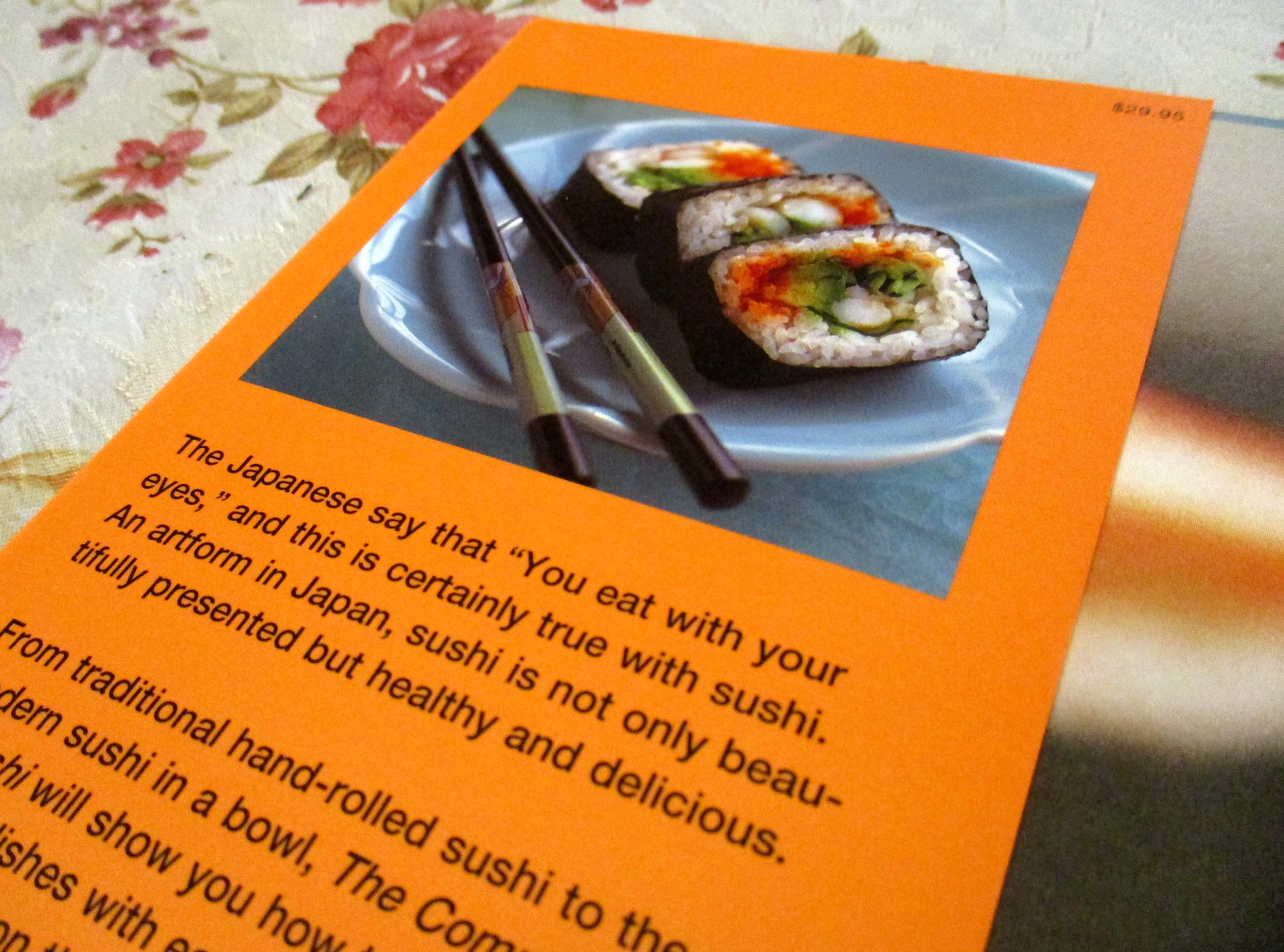The photograph captures an orange placard, likely the back cover or promotional sheet for a book on sushi, displayed at a tilted angle. The placard rests on a white tablecloth adorned with a red rose, adding delicate floral detail to the setting. The top part of the orange placard showcases a white plate with two chopsticks and three pieces of sushi, elegantly arranged to highlight the artistry of Japanese cuisine. Beneath this image, black text reads: "The Japanese say that you eat with your eyes, and this is certainly true with sushi. An art form in Japan, sushi is not only beautifully presented, but healthy and delicious." Though the text is partially cut off, fragments suggest it describes various types of sushi, including traditional hand-rolled sushi and modern sushi bowls. To the left of the placard, a floral-patterned placemat is visible, and the right edge of the photo features an out-of-focus section that might be part of a menu, hinting at a price of 29.95.